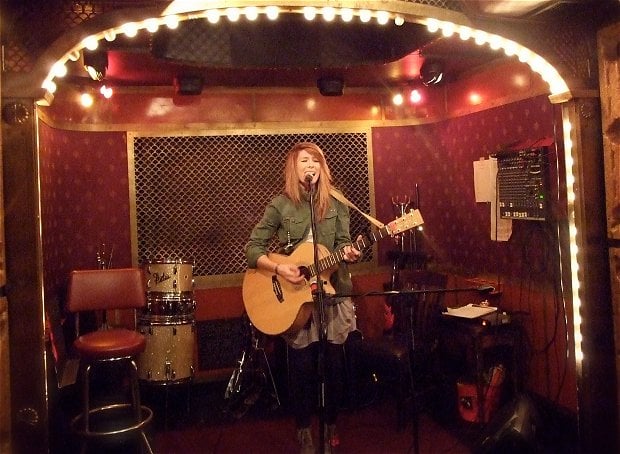In this vibrant color photo of an intimate interior space, we see a small stage glowing with yellow lights that border the ceiling edge and the stage. Dominating the scene is a young woman, likely in her twenties, with long reddish-brown hair and fair skin. She is at the center of the stage, passionately singing into a microphone. 

She stands confidently, dressed in an olive green long-sleeve shirt paired with a white skirt layered over black yoga pants. Cradling an acoustic guitar with a traditional brown finish, she wears a strap over her shoulder as she performs. 

To her right, there's a high silver-framed stool with a reddish-brown back and seat, adding to the stage's cozy aesthetic. Behind her, a snare drum and bass drum subtly hint at the musical atmosphere. The room itself exudes a warm, red hue, enhancing the inviting and unique ambiance of this musical moment.